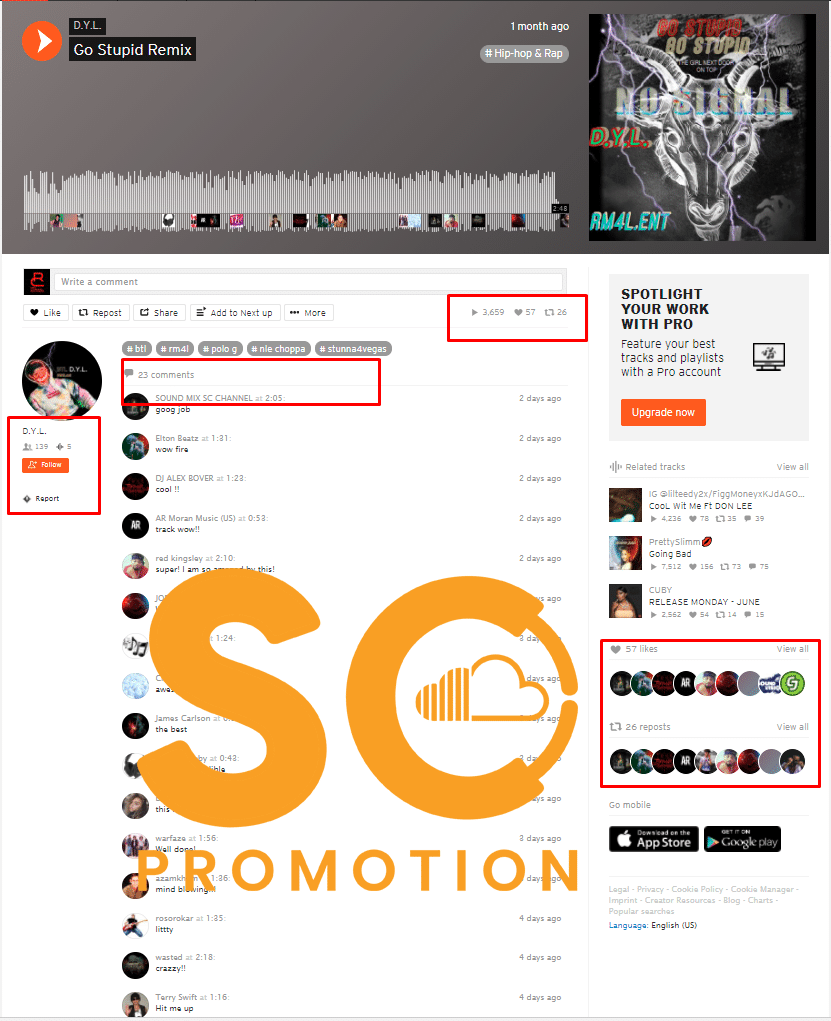The image is a screenshot featuring a music streaming platform interface, highlighting a track titled "Go Stupid Remix" by D.Y.L. At the top, a dark gray bar displays the track name, genre (Hip Hop & Rap), and the upload timestamp (one month ago). On the right side of the screen, there is an album cover depicting a goat skull with horns, labeled "Go Stupid No Signal D.Y.L. R.M.4L.E.N.T."

To the left of the album cover is a white bar graph, signifying the audio file. The main section of the website has a white background and is labeled "S.O. Promotion." Below this, there is a comment section where users can leave comments. The user D.Y.L. has options to be followed, reported, or spotlighted, marked by a red square around the follow and report buttons. 

In the middle, a red square highlights "23 comments," and another red rectangle draws attention to the number "3,659," likely indicating plays or views. Additionally, 57 people have favorited the track, and 26 people have retweeted it. On the right-hand side, a promotional message encourages users to "Spotlight your work with Pro," urging them to upgrade to a Pro account to feature their best tracks and playlists.

Further down, more tracks are listed, and a red rectangle surrounds "57 likes, view all" and "26 reposts, view all," summarizing the track's interaction metrics.